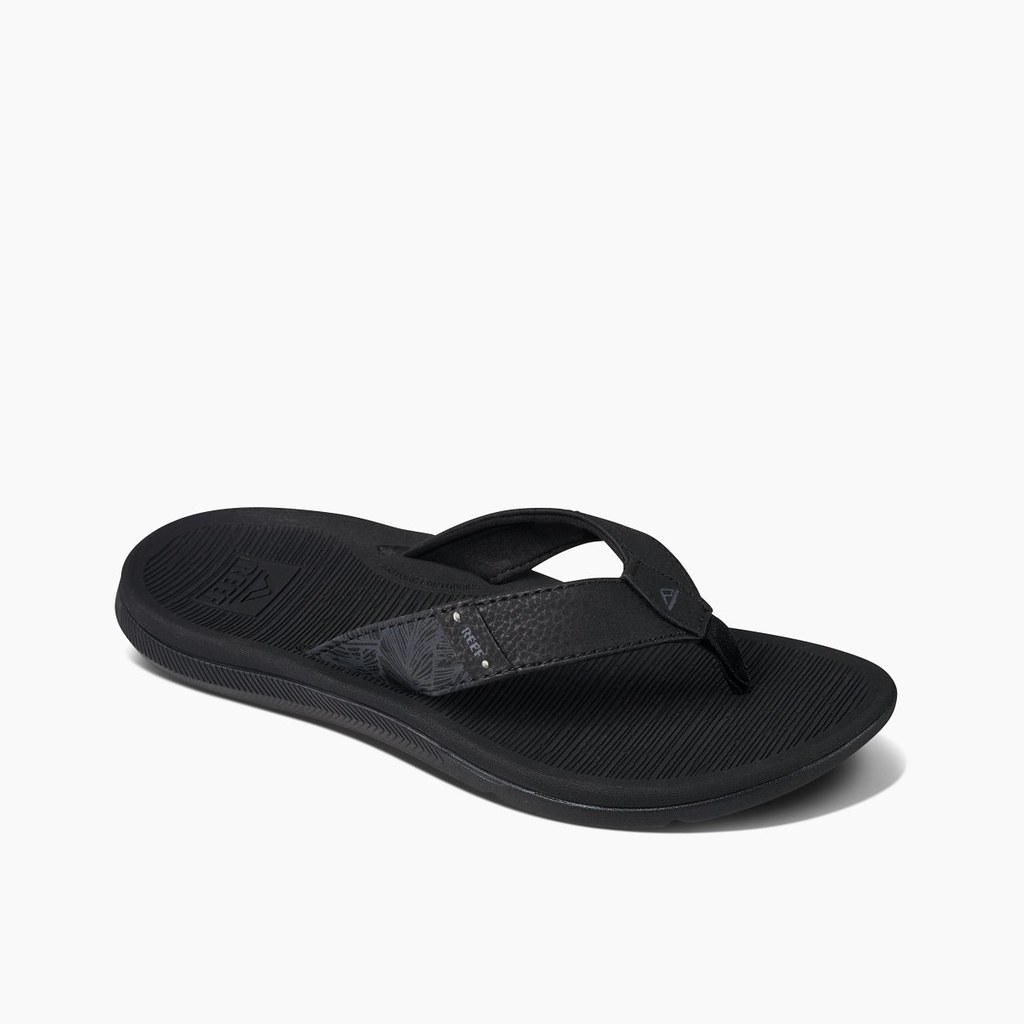This image features a single right-foot sandal positioned slightly lower than the center of a vertical rectangular photograph. The sandal, predominantly black, contrasts sharply against the crisp white background, which helps draw focus to its details. The sandal has a flip-flop style design, with a medium thickness black rubber sole that exhibits horizontal ridges. Additionally, it features a black leather strap adorned with subtle patterns and a small vertical rectangular logo on the right strap. This logo, fastened with two silver circles, displays the brand name "REEF" in gray capital letters. An intricate gray plant pattern can also be seen near the toe area, enhancing the overall design of the sandal. A slight shadow of the sandal is visible on the white surface, adding depth to the image.